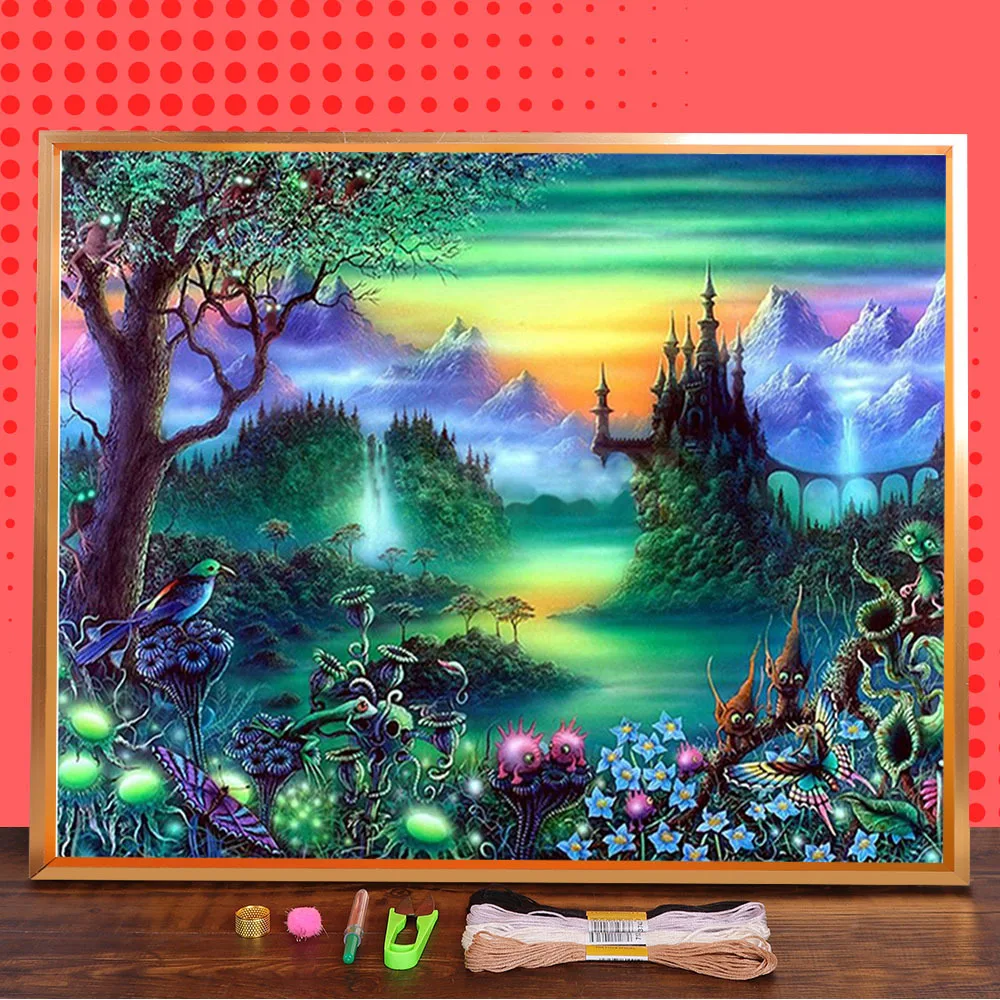This photo showcases a framed, vividly colored fantasy artwork, encased in a plain, thin brown wooden frame. The centerpiece of the print is a radiant green water body surrounded by lush greenery. In the distance stands an island featuring an elaborate castle, majestically connected by a large arched bridge. In the foreground, whimsical plant-like creatures, two of which are brown, gaze in awe at a large butterfly. The lower left corner is adorned with striking blue and green flowers, hosting a small frog and a bird perched among them. A towering tree on the left side is home to monkey-like creatures with large, glowing eyes. The background is completed with imposing purple mountains, all under a mesmerizing, multicolored sky painted in hues of green, yellow, and orange.